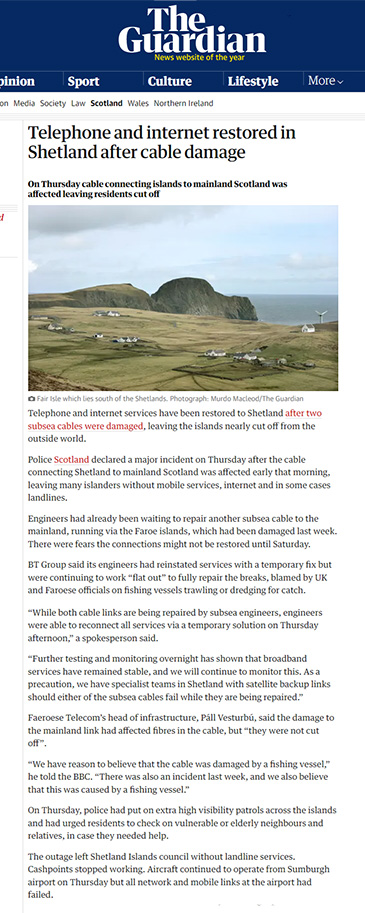In this image, we see a screenshot of an article from The Guardian. At the top of the page, "The Guardian" is prominently displayed in large white letters. Directly below the title, there are clickable options leading to various sections: "Opinion," "Sport," "Culture," "Lifestyle," and "More," which provide access to articles in these categories. 

The headline of the featured article reads, "Telephone and Internet Restored in Shetland After Cable Damage." The subheading details that on Thursday, a cable connecting the Shetland Islands to mainland Scotland was damaged, resulting in the residents being temporarily cut off from communication services. 

Accompanying the article is a picturesque photograph of the town of Shetland, showcasing its coastal beauty. Beneath the image, there is a continuation of the article that delves deeper into the incident and the restoration efforts.